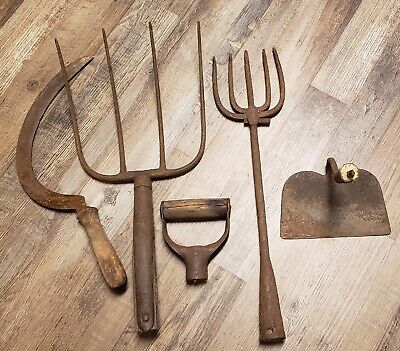This color photograph, presented in a square format, captures a collection of vintage gardening and farming tools lying side-by-side on a diagonally aligned, shiny beige-brown wooden floor. The well-used tools, characterized by their rusted metal and rich patina, suggest a history of long and diligent use. From left to right, the lineup includes a hack, a four-pronged fork, a detached handle believed to belong to the fork, a slender five-pronged pitchfork, and the metal scoop of a shovel. The centerpiece of the arrangement is a larger hay pitchfork. Two of the items, the handle in the center and the hoe on the right, notably lack their wooden dowels. The photograph embraces a style of photographic representational realism, emphasizing the textured details and aged appearance of the tools against the pristine wooden background.